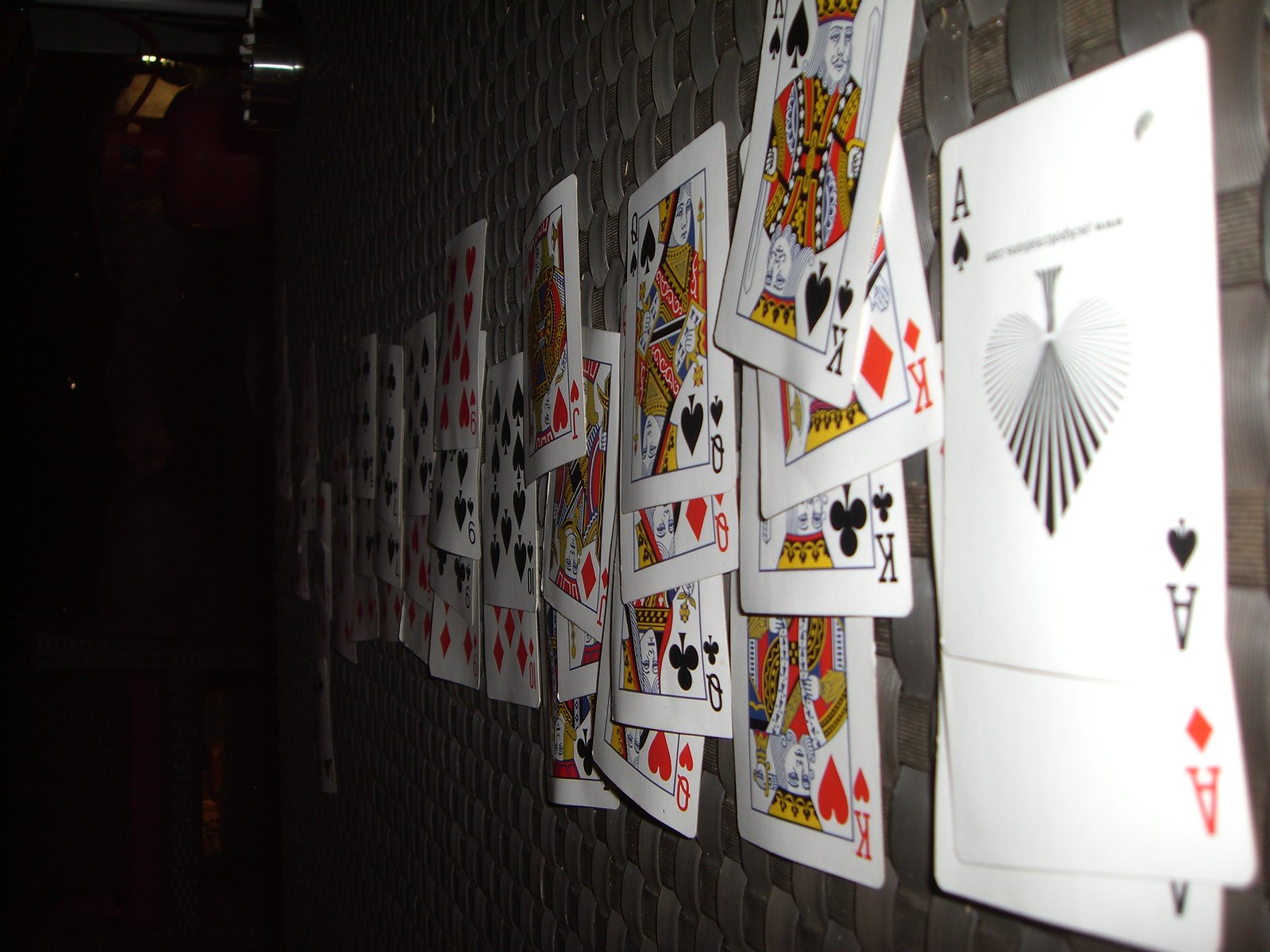This photograph captures an outdoor table woven from what appears to be palm leaves or bamboo. The surface of the table is taken up by a meticulously arranged game of solitaire. The camera angle is unique, lying close to the table, offering an intimate and detailed perspective of the tableau. There are approximately 15 rows of cards, each with three or four cards stacked neatly on top of each other. 

On the right side, the tableau starts with a series of aces: the Ace of Clubs, Ace of Diamonds, and likely Ace of Spades and Ace of Hearts, setting up the foundation for the game. Following the aces, in descending order, are the Kings of Spades, Diamonds, Clubs, and Hearts, then the Queens, Jacks, and so on, each rank arranged in its own stack, gradually decreasing in value.

The background of the image is shrouded in darkness, suggesting that the photograph was taken without a flash and in a dimly lit area. The quality of the image is somewhat poor, with the dark background contributing to the lack of clarity. Despite this, the intricate details of the cards and the woven texture of the table are still discernible, highlighting the careful setup of the solitaire game in this outdoor setting.